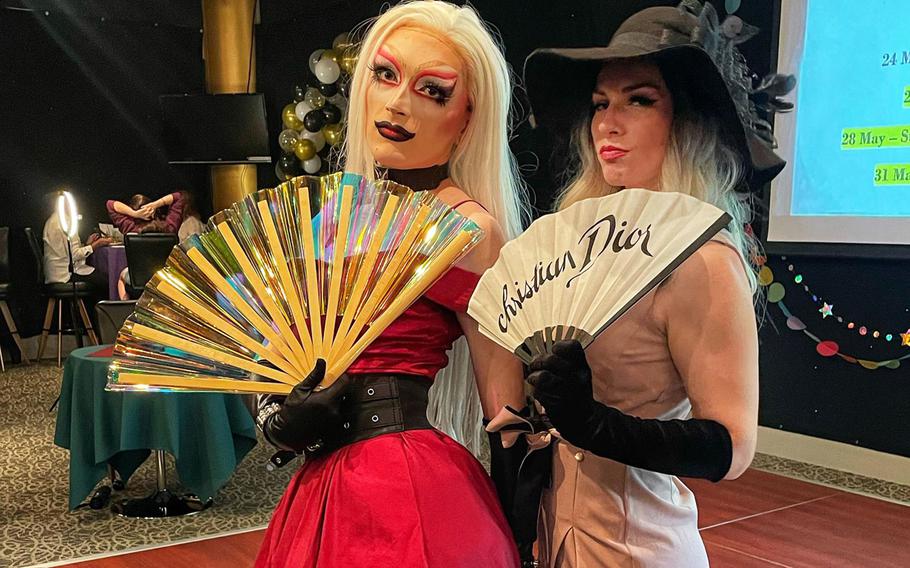In this photograph, set in what appears to be a convention center, two elaborately dressed drag queens pose prominently in the foreground. The drag queen on the left is adorned in an off-the-shoulder red dress, cinched at the waist with a wide black cummerbund. She wears a long platinum blonde wig and black opera gloves, her makeup is striking with black and red accents around her eyes, and she holds a large, iridescent gold fan. To her right, another drag queen is dressed in a tan dress accompanied by black elbow-length opera gloves and a wide-brimmed black hat. This queen also sports a blonde wig and holds a fan emblazoned with the name "Christian Dior." Both figures, with their dramatic makeup and striking attire, give the impression of wax museum sculptures. 

In the background, a balloon arch composed of black, gold, and silver balloons adds a festive touch, while a table covered with a green tablecloth can be seen. Further behind, two men are visible; one appears to be lounging with his hands on his head, while the other is seated, possibly at a table or some unknown object. A portion of a projector screen is also visible, displaying dates in black lettering: "24, 28 of May through 31st of May." This detailed backdrop suggests the photograph was taken at a lively event or convention.